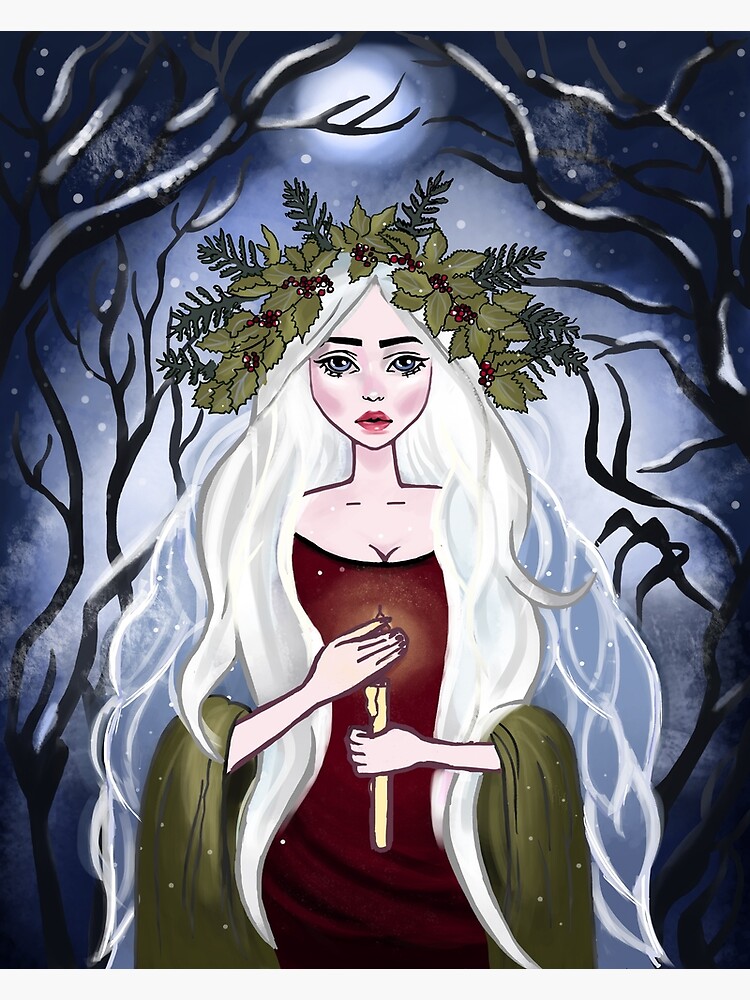In this striking winter scene illustration, a woman with very long, flowing white hair stands outdoors under a clear, moonlit sky. Her pale complexion and large, open eyes create a serene yet captivating presence. She wears a rich, reddish-burgundy dress over which a long, green shawl is draped, cascading elegantly around her back and forearms. Atop her head is a detailed wreath of holly leaves and red berries, adding a touch of earthy elegance. In her hands, she holds a tall, tapered candle, shielding its flame with her right hand while gripping it firmly with the other. The candle shows signs of melting, with wax delicately dripping down its sides. The background features bare, stylized black trees edged with snow, set against a dark, blue night sky where snowflakes gently fall. The full moon glows softly overhead, casting a tranquil light that enhances the ethereal atmosphere of the scene.